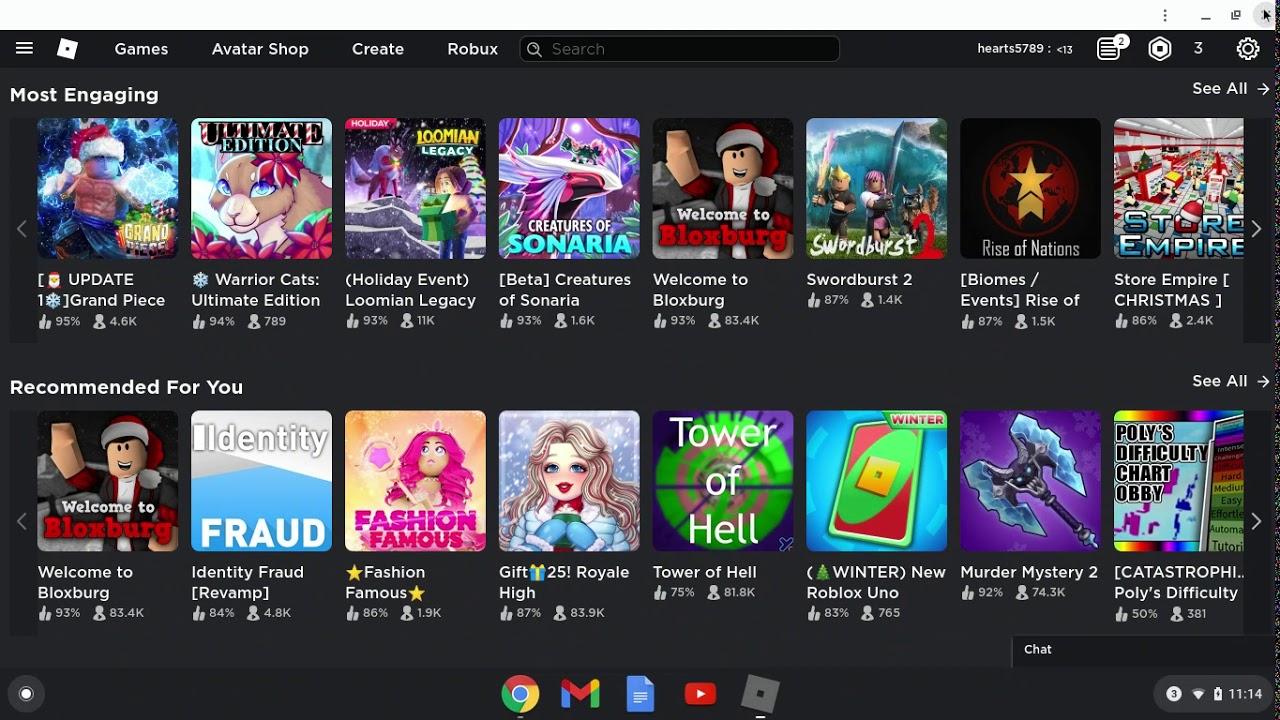A screenshot depicts a game shop interface on what appears to be a desktop environment. The top border is white, featuring several icons on the far right: three stacked horizontal dots, minimize window, expand window, and a close window 'X,' over which the black arrow cursor hovers.

Below the top bar, the program's interface features a black background. In the upper left corner, there are three horizontal lines, followed by a white square with a black dot, and then the text options "Games," "Avatar Shop," "Create," and "Robux," all in white. To the right, a black search bar with a white magnifying glass icon and the word "Search" is positioned. Further right, a username "hearts5789" (in lowercase letters) is displayed in white text, accompanied by an arrow and the number 13. Adjacent to that is a document icon with lines and a white circle bearing the number 2, followed by a white cube, and a gear icon showing the number 3.

In the lower-left corner, the section titled "Most Engaging" (both words capitalized) is displayed, and on the far right of this section, the "See All" option with a right-pointing arrow is visible. Below these titles, there are images and titles of games with corresponding engagement statistics from left to right:

1. "Update Grand Piece" – 95% thumbs up, 4.6K plays.
2. "Warrior Cats Ultimate Edition" – 94% thumbs up, 789 plays.
3. "Holiday Event: Lumion Legacy" – 93% thumbs up, 11K plays.
4. "Beta Creatures of Sonaria" – 90% thumbs up, 1.6K plays.
5. "Welcome to Bloxburg" – 93% thumbs up, 83.4K plays.
6. "Shindo Life" – 87% thumbs up, 1.4K plays.
7. "Biomes Events: Rise of Nations" – 87% thumbs up, 1.5K plays.
8. "Store Empire: Christmas" – 86% thumbs up, 2.4K plays.

Further down, in the left-middle section, there's a "Recommended for You" section with the following games listed:

1. "Welcome to Bloxburg"
2. "Identity Fraud: Revamped" – 84% thumbs up, 4.8K plays.
3. "Fashion Famous" – 86% thumbs up, 1.9K plays.
4. "Day 25 Royale High" – 87% thumbs up, 3.9K plays.
5. "Tower of Hell" – 75% thumbs up, 81.8K plays.
6. "Winter New: Roblox Uno" – 83% thumbs up, 765 plays.
7. "Murder Mystery 2" – 92% thumbs up, 74.3K plays.
8. "Catastrophic Polly's Difficulty Chart Obby" – 50% thumbs up, 381 plays.

At the bottom, the chat window is labeled "Chat" in white text. Additional interface elements include a white circle in the bottom left, icons for Chrome, Gmail, Google Docs (a blue document), YouTube, and a gray box. On the bottom right, there’s a white circle with the number 3, a Wi-Fi signal icon, a battery icon, and the current time displayed as 11:14.